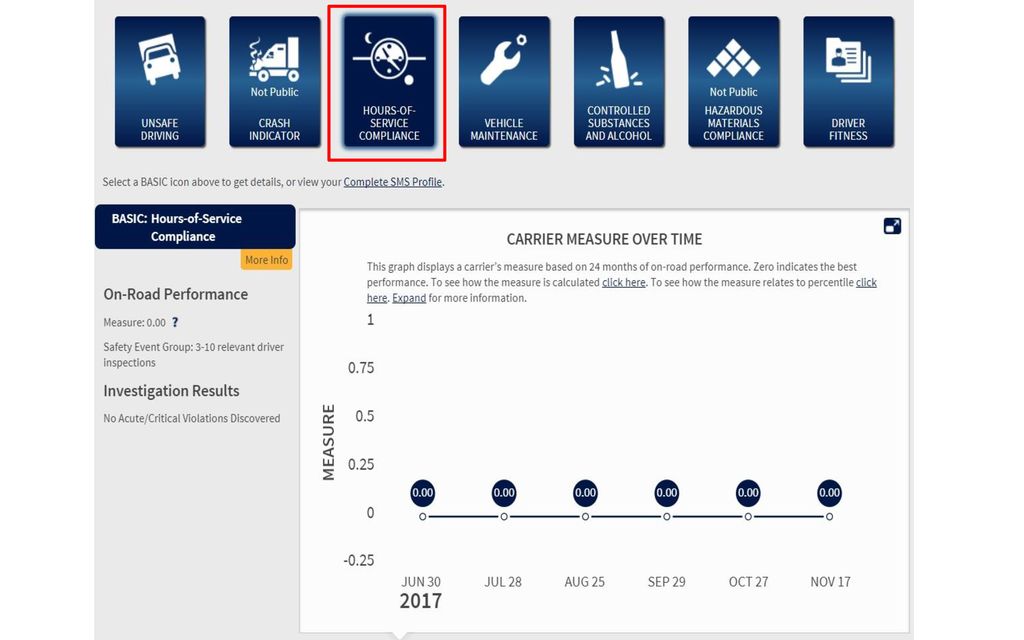The image depicts a detailed interface of a safety compliance website. The layout includes a light gray background on the left and the name of the website at the top. At the top of the interface, there is a row of seven square icons, each surrounded by a navy blue border on the top and bottom, and a slightly lighter blue in the center. 

Each square represents a different safety compliance category:
1. Unsafe Driving
2. Crash Indicator
3. Hours of Service Compliance (highlighted with a red outline)
4. Vehicle Maintenance
5. Controlled Substances and Alcohol
6. Hazardous Materials Compliance
7. Driver Fitness

Below this row of icons, a navy blue banner prominently displays the text "BASIC: Hours of Service Compliance," indicating the main focus. Beneath this, a yellow-orange banner provides additional information titled "More Info: On-Road Performance Investigation Results."

To the right, an off-white background section features a graphical representation titled "Carrier Measure Over Time," showing metrics tracked over several months. The y-axis is labeled "Measure," while the x-axis details specific dates: June 30, 2017, July 28, August 25, September 29, October 27, and November 17.

This thorough layout visually organizes important compliance and performance data to assist in monitoring and evaluating safety measures.